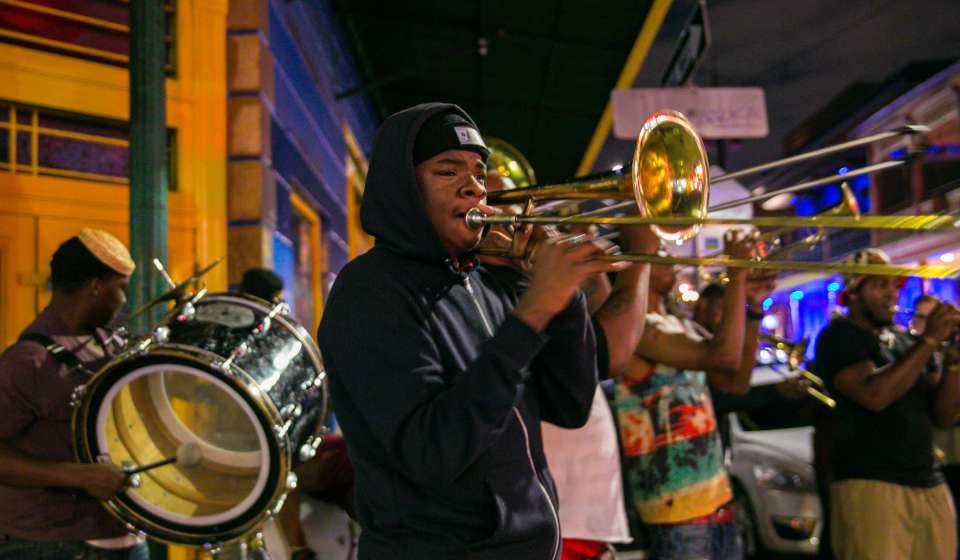In this vibrant photograph, a lively street band is performing on a bustling corner, likely in New Orleans. The band consists of five members, with a diverse array of instruments and attire that contribute to the vivid atmosphere. 

In the lower left corner, a drummer with a portable drum featuring transparent membranes adds rhythm to the scene. The focal point of the image is a black man in the center, dressed in a blue jacket, hoodie, and cap, who is passionately playing the trombone. To his left stands another musician in a white shirt and red pants, energetically playing a trumpet. Next to him is a bandmate donning a colorful tie-dye shirt, also engrossed in playing a horn. To the far right, a man in a black shirt and tan pants joins in with his own trumpet, completing the harmonic ensemble.

The background is equally lively, with colorful buildings in shades of yellow, blue, brown, green, and orange adding to the festive ambiance. A parked white car can be seen behind the band, along with more urban elements like an overpass and various pedestrians watching the performance. This scene captures the essence of New Orleans' rich musical culture and its vibrant street life.